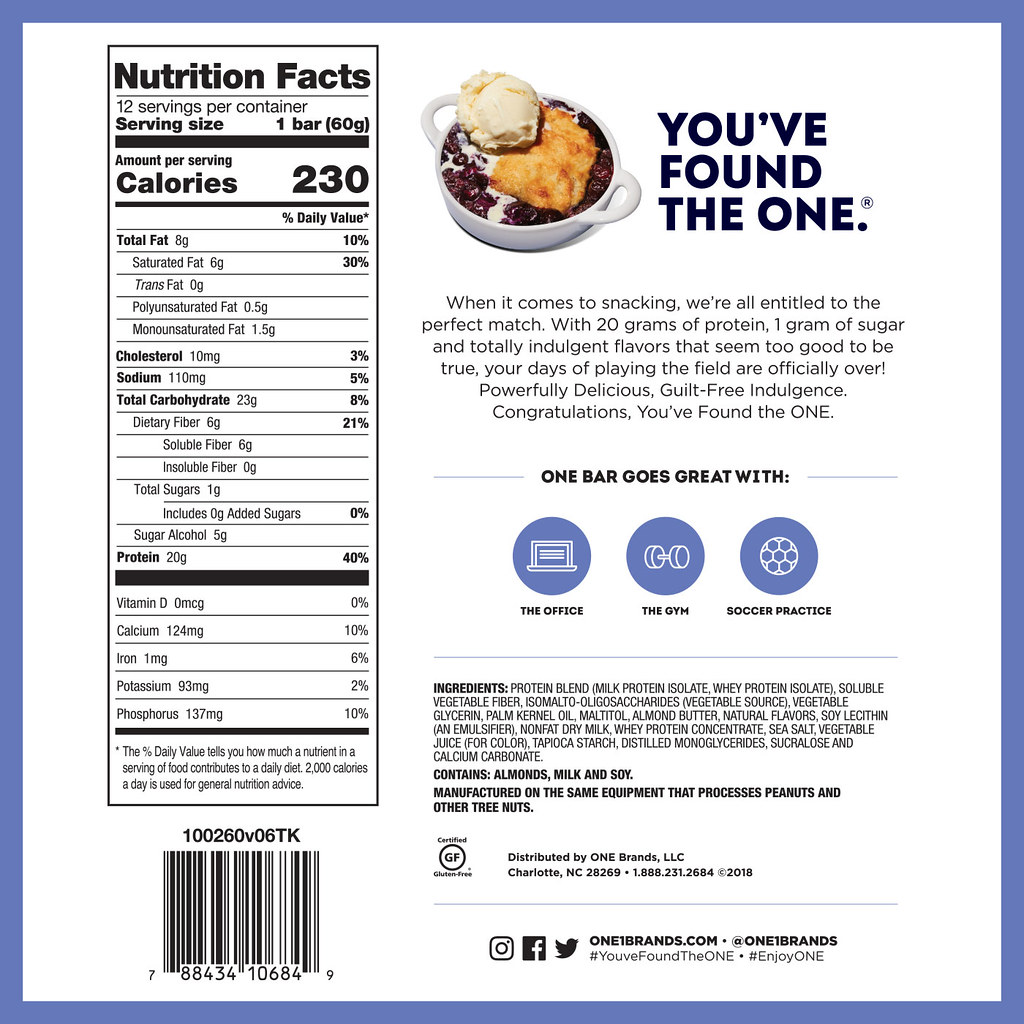**Caption: Detailed Product Information for One Bar**

The image features the complete product information for a nutritional bar. On the left side, it presents detailed nutrition facts, indicating there are 12 servings per container, with each serving being one bar. Each bar contains 230 calories alongside information on fats, cholesterol, and other nutritional values, including their respective percentages of the daily recommended intake. At the bottom of the nutrition facts section, the UPC code is visible.

On the right side of the image, a vivid photograph showcases a white bowl with handles on both sides. The bowl is filled with cranberries, ice cream, and pieces of the bar. Above this, bold text reads, "You found the one." The accompanying description states, "When it comes to snacking, we're all entitled to the perfect match. With 20 grams of protein, one gram of sugar, and totally indulgent flavors that seem too good to be true, your days of playing the field are officially over. Powerfully delicious, guilt-free indulgence, congratulations, you found the one." Additionally, it mentions that the bar pairs perfectly with activities like office work, gym sessions, and soccer practice.

Further down, there is a comprehensive list of ingredients and information about the manufacturer, all set against a background bordered by a blue edge.